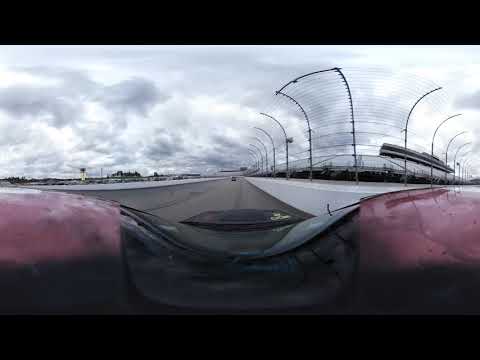The image depicts a first-person view from inside a red race car driving on a racetrack during an overcast day, with dark gray and white clouds filling the sky. The fisheye perspective captures the expansive gray asphalt track that loops around a large stadium area, which appears to be completely empty with no spectators present. To the right and left of the track are tall metal fences, approximately 15 to 20 feet high, designed to protect the audience, though the stands are vacant. Concrete barriers line both sides of the track to keep the cars contained. In the middle distance, there are some buildings visible on the left side, and a car far ahead of the driver. The image also shows reflections on the hood of the red car, enhancing the dramatic and intense atmosphere of the racetrack setting. There is a large parking lot visible within the infield area of the track, filled with cars, emphasizing that the race is taking place during daytime under a sky heavily laden with dark, brooding clouds.